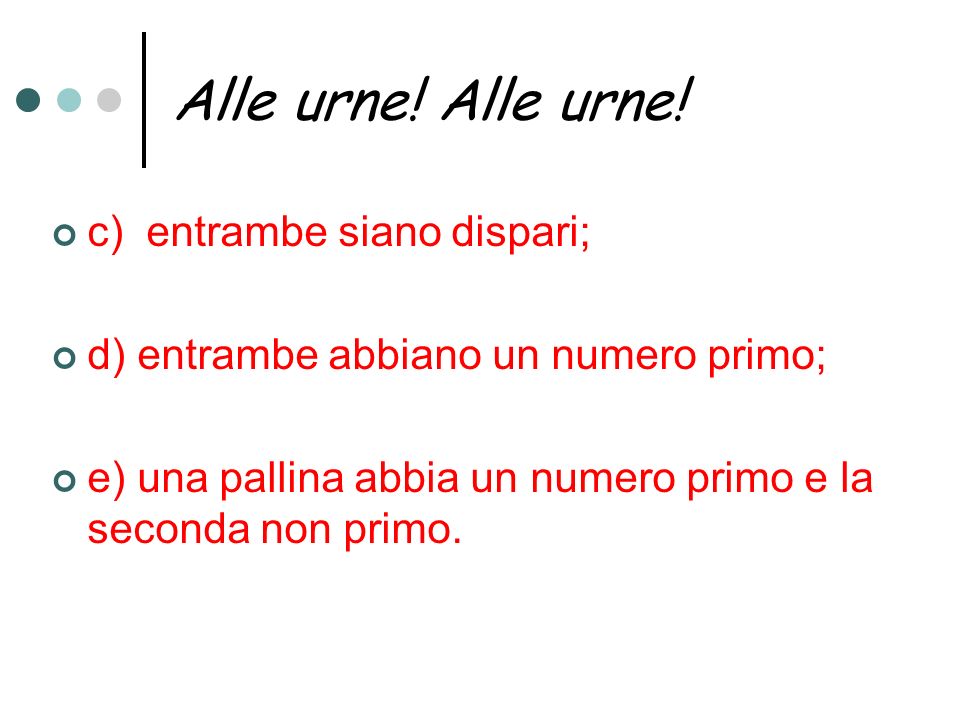The image features a white background with two lines of black text at the top, each reading “A-L-L-E-U-R-N-E!” with exclamation points following each instance. To the left of this text are three dots: the first is green, the second is a lighter green, and the third is gray. Below the title, three sections are indicated by light green bullet points labeled C, D, and E, each containing text in red font, which appears to be in Italian. Section C reads "Entrambe Siano Dispari," section D reads "Entrambe Aviano Un Numero Primo," and section E reads "Una Palina Avia Un Numero Primo E La Seconda Non Primo." A vertical line separates the dots from the title text, emphasizing the structured layout.